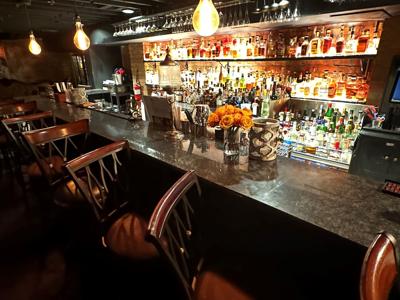This image captures the interior of an empty bar, showcasing a sleek and shiny, long rectangular bar counter that appears black. The bar, set on an angle from right to left, features five to six barstools, each with a round, brown seat and backrests framed in shiny wood. Above the bar, three large yellow light bulbs hang from the ceiling, illuminating the scene with a warm glow.

On the bar counter, there's a vase filled with bright orange flowers, adding a pop of color to the predominantly dark and brown-hued setting. Additionally, various bottles can be seen on the counter, contributing to the bar's detailed ambiance.

Behind the bar, the illuminated brown wall is lined with three mirrored shelves, each filled with a vast array of liquor bottles, reflecting a soft, glowing light. The entire atmosphere of the bar is highlighted by the symmetry and shine from both the glass shelves and the bottles, creating a striking visual effect. The overall mood is dark yet warm, accentuated by the brown and yellow tones, and the absence of people lends it a tranquil, almost serene quality.